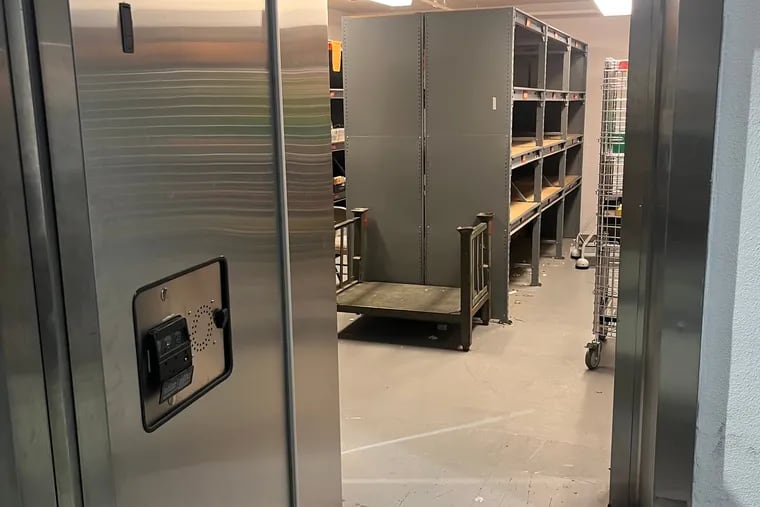This photograph depicts a room that appears to be some type of storage area or possibly a refrigerated section. The predominant color scheme is gray and silver, giving the room a sleek, stainless steel look. The floor and walls are gray, and the room is brightly lit with long, rectangular fluorescent lights on the ceiling. 

You can see into the room through a silver door that has a small speaker panel and a black panel on it. Inside, there are several empty, silver metal shelves lining the walls, contributing to a spacious but stark atmosphere. To the right, there is a rolling metallic cage with wheels, and further inside, there is another rolling cart. On the left, there is a low-to-the-ground, four-legged metal bench or rack. The overall scene captures an organized but currently unused storage space with a cold, industrial feel.